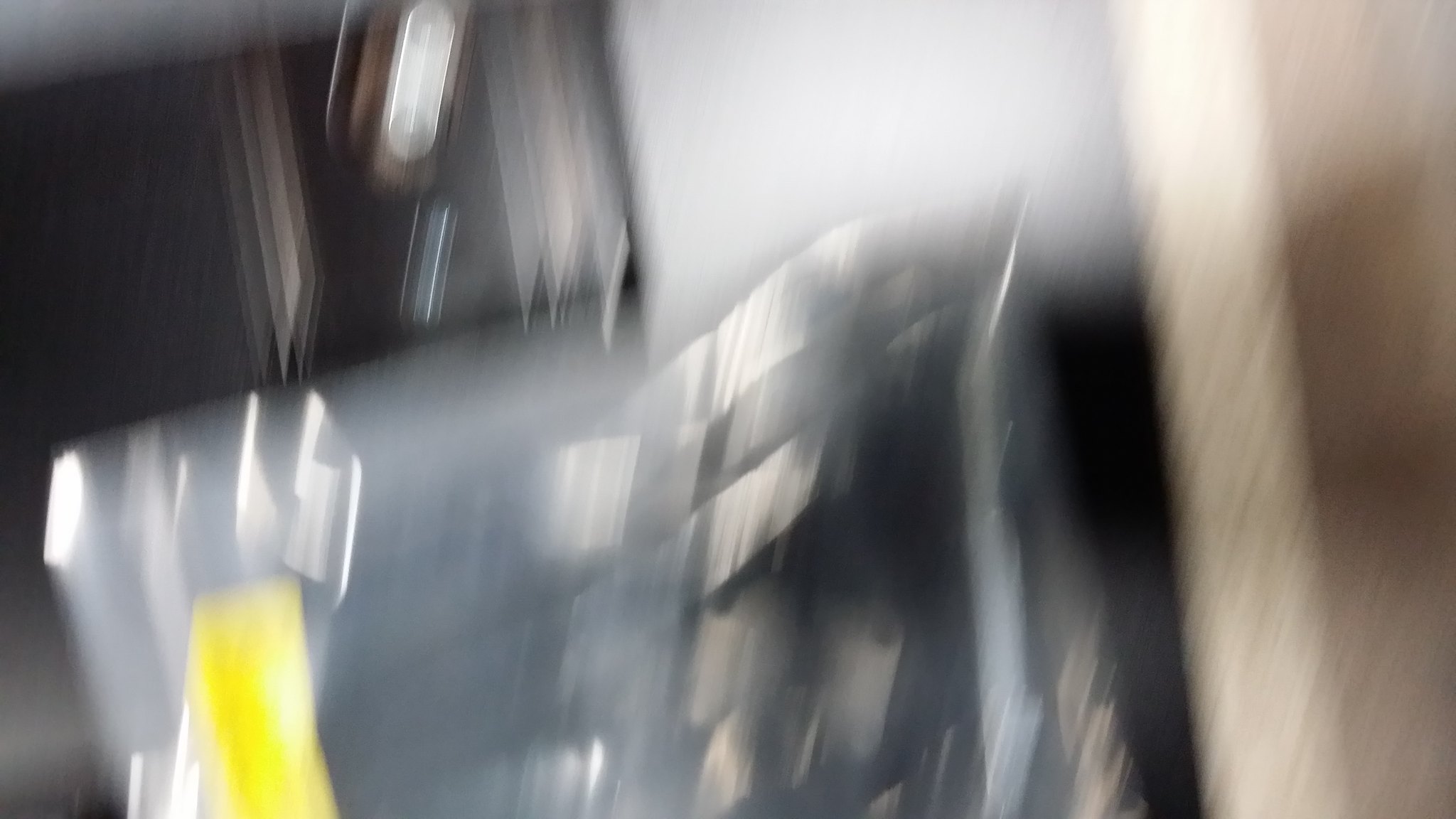This horizontal photograph is dominated by a pronounced blur, making it challenging to identify specific objects within the frame. In the lower right portion, a dark, curved structure resembling the front of an automobile—complete with a bumper, headlights, and a grille—can be faintly discerned. Adjacent to this, a white rectangular shape spans the right edge, suggesting illumination from some light source. The upper central area features a light gray patch that contrasts the surrounding darkness. On the left, a bright white rectangular form seems to be directing sunlight or intense white light downward onto the ambiguous, dark forms below. On the lower left, there is another rectangular object, marked by a yellow body and a white top. Despite these identifiable elements, the overall blurriness and lack of detail render the true nature of the scene indeterminable.